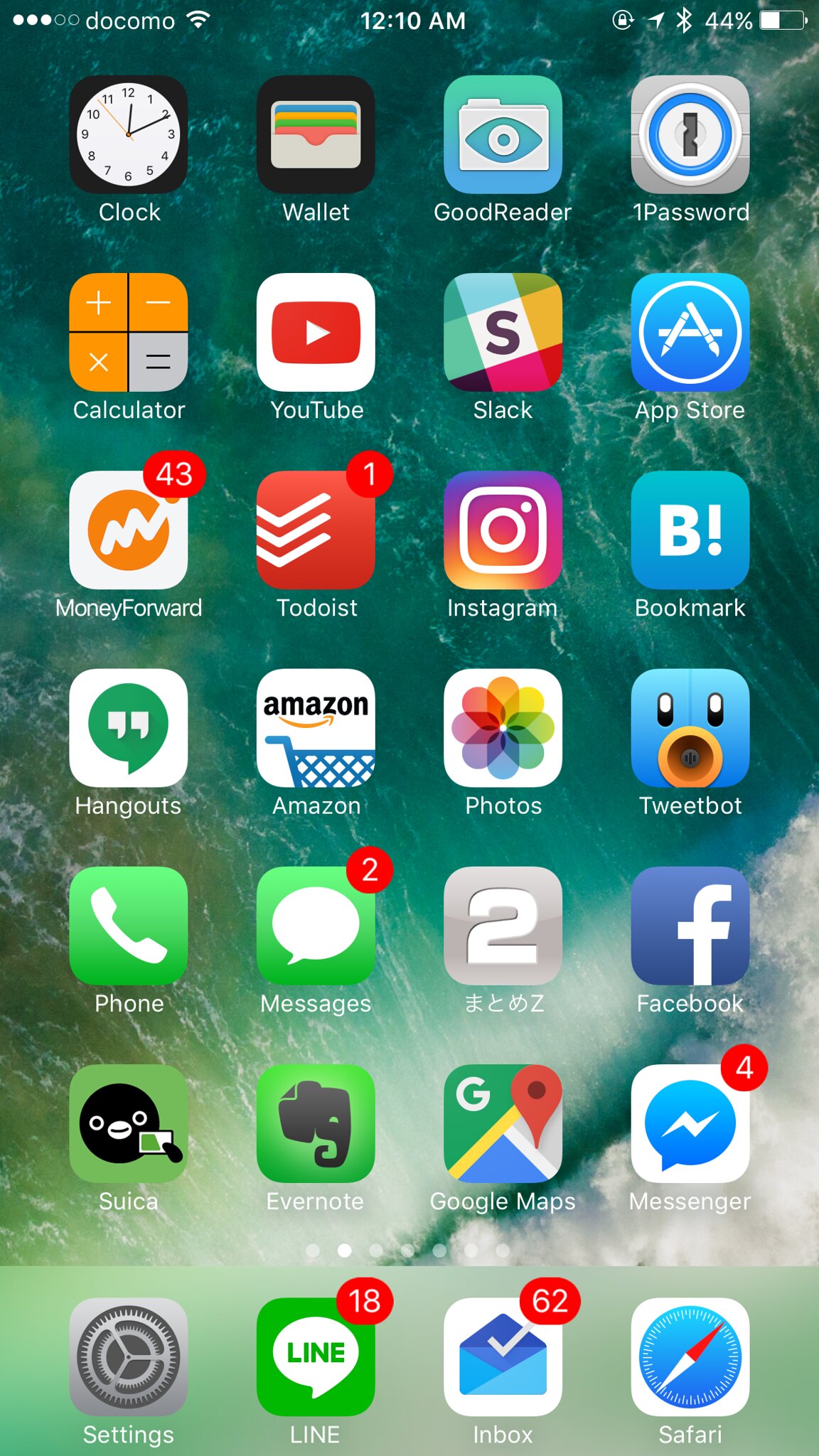This is a detailed screenshot of a smartphone's home screen. At the top left, there are five dots indicating signal strength, with three filled in white and two remaining clear. Adjacent to these dots, the carrier name "Docomo" is displayed, followed by a Wi-Fi symbol. Centered at the top is the current time, "12:10 AM." On the top right, there is a sequence of icons including a circle with a lock, a GPS symbol, a Bluetooth symbol, and the battery charge represented as "44%" accompanied by a battery icon.

The main section of the home screen showcases 24 app icons arranged neatly in a grid format. Below these app icons, the dock contains four additional applications: Settings, Line, Inbox, and Safari, indicated by their respective icons. Above the app grid, there is a row of seven navigation dots with the first one filled in white, highlighting the current home screen page, while the rest are clear.

The background image depicts a scenic view of water with gentle waves, adding a serene aesthetic to the home screen.